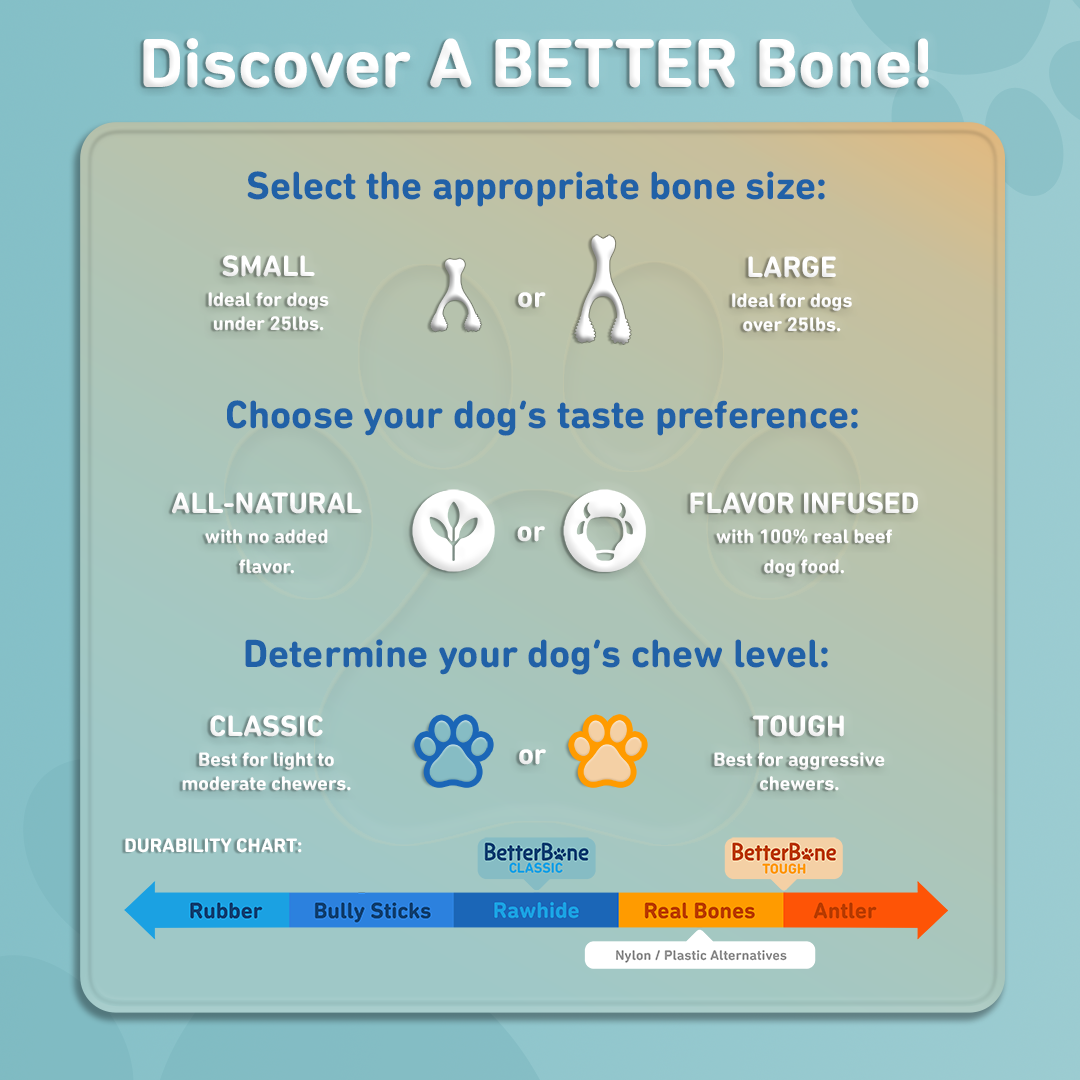The image is a detailed, 3D-style diagram with a predominantly blue background featuring paw prints, aimed at helping dog owners select the appropriate bone for their pets. At the top of the diagram, white bold text states, "Discover a Better Bone." Below this, a section titled "Select the Appropriate Bone Size" features small and large bone options—small is ideal for dogs under 25 pounds and large for dogs over 25 pounds. The next section, "Choose Your Dog's Taste Preference," offers options of all-natural bones with no added flavor or flavor-infused bones with 100% real beef. This is visually represented by plant and cow logo icons. The following section, "Determine Your Dog's Chew Level," has blue and yellow paw prints indicating "Classic" for light to moderate chewers and "Tough" for aggressive chewers. Toward the bottom, a "Durability Chart" spans from blue (rubber) to red (antler), showing the ranking of their bone options—Better Bone Classic and Better Bone Tough—relative to other materials. The chart helps dog owners decide the most suitable bone type based on their dog's chewing needs.